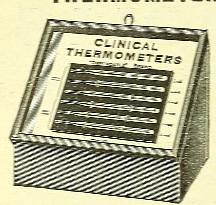This vintage, zoomed-in photograph, likely clipped from an old newspaper or news article, depicts a clinical thermometer prominently displayed in a glass case. The thermometer is housed in an intriguingly designed box, which rests at an angle, creating a visually striking presentation. The front part of the box is shorter, while the back stands about twice as high, giving the box a tilted, plaque-like appearance. Underneath the heading "Clinical Thermometer," six distinct lines of text are visible, though no additional words can be discerned from the image. Diagonal lines decorate the lower portion of the box, adding to its detailed design. Enclosed behind glass, this clinical thermometer appears to have been a historically significant, well-preserved medical tool, once advertised with pride.